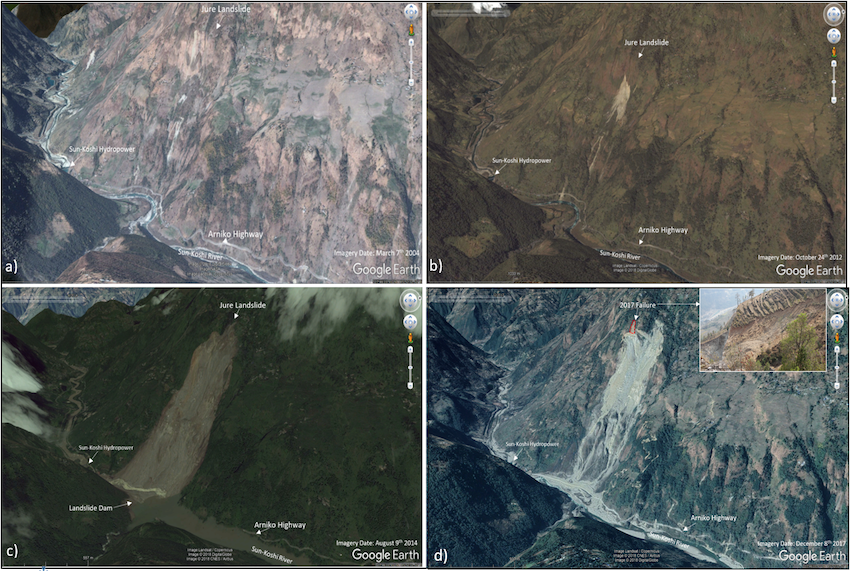The image composition consists of four Google Earth snapshots arranged in quadrants: upper left, upper right, lower left, and lower right. Each of these equal-sized images captures a distinct location and appears to document the Jure Landslide over time. The upper left image, labeled with the date 2004, shows a mountainside characterized by various colors such as pink, gray, darker gray, brown, and green, indicating diverse terrain and possible vegetation; the presence of a highway is also noted. The upper right image seems to depict a desert landscape with sandy terrain and visible cracks. The lower left image features a highway, cloud cover, and a mountainous region, while the lower right image presents a waterfall. The waterfall cascades down a mountain adorned with gray rocks and green moss, leading to a stream surrounded by trees. Small text annotations in each quadrant describe the landmarks and the specific events, indicating the dynamic changes in the landscape over time, with a particular focus on the Jure Landslide.